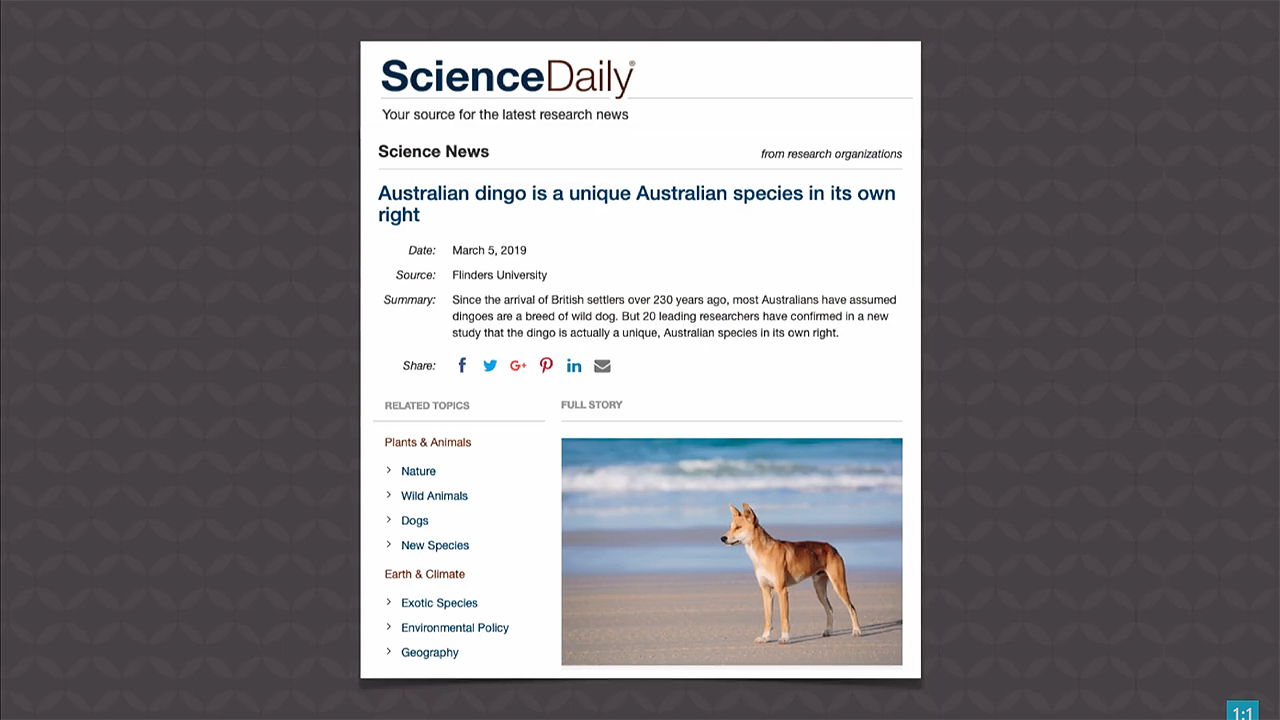On a mid-gray diamond-patterned background, the top section features a white banner with the word "Science" in blue, followed by "Daily" in brown. Beneath this header, a thin black line separates it from the tagline, "Your resource for the latest research news," in black text. Below, the title "Science News" appears in bold black, accompanied by the italicized phrase "from research organizations," separated by a thin gray line. 

The main headline, in bold blue, announces, "Australian dingo is a unique Australian species in its own right." The date, "March 5th, 2019," is displayed in regular black text, labeled "Date" in italicized black. The source, "Flinders University," is also presented in regular black, prefixed by the italicized label "Source." 

The summary, marked by the italicized word "Summary," states, "Since the arrival of the British settlers over 230 years ago, most Australians have assumed dingoes are a breed of wild dog. But 20 leading researchers have confirmed in a new study that the dingo is actually a unique, Australian species in its own right."

Social media icons appear below, including a blue Facebook 'F', a light blue Twitter bird, a red Google+ 'G' and '+', a maroon red Pinterest 'P', a dark blue LinkedIn 'in', and a dark gray envelope icon for email.

The section titled "Related Topics" in gray is followed by a gray line, and the categories "Plants and Animals" in bold red text. Dark gray right-pointing arrows lead to subtopics in bold blue text: "Nature," "Wild Animals," "Dogs," "New Species." Following this, "Earth and Climate" appears in bold red, with more subtopics: "Exotic Species," "Environmental Policy," and "Geography," again connected by dark blue arrows.

On the right-hand side, the image of a dingo stands on a beach with bands of brown and tan sand, reflecting shades of blue from the waves and sky. Snow-capped waves crash towards the wet, water-flooded beach, displaying a mixture of teal, dark blue, and cyan water. The dingo, mostly tan with sporadic brown spots, looks to the left, featuring black markings around its nose and mouth, perky pointy ears, and eyes encircled by black.